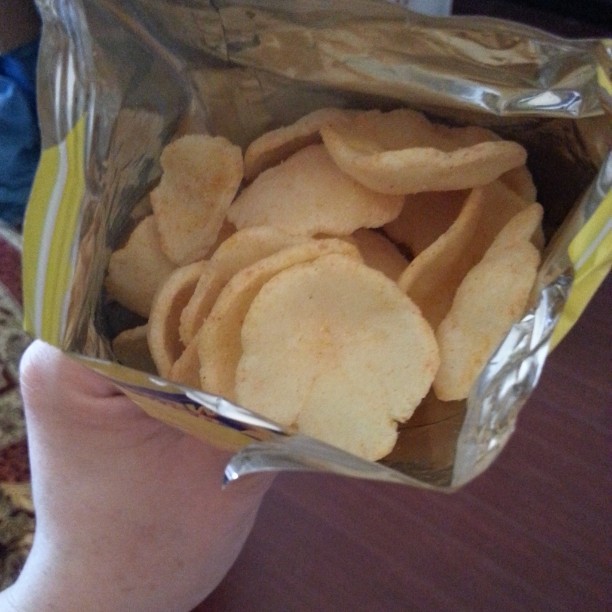This is a poorly lit, top-down photograph showing an open bag of crispy snacks held by someone's left hand. The inside of the bag is metallic silver, while the outside features a combination of yellow, white, and blue colors. The bag rests above a brown wooden floor, which is barely visible. The snacks inside are irregularly shaped, somewhat circular, and exhibit a pale beige or orangey hue, suggesting they might be seasoned. Their exact type is unclear, but they resemble potato or fish crisps, potentially like those from the Oishi brand. Despite the image quality being subpar, the thick, crunchy texture of the snacks is discernible.